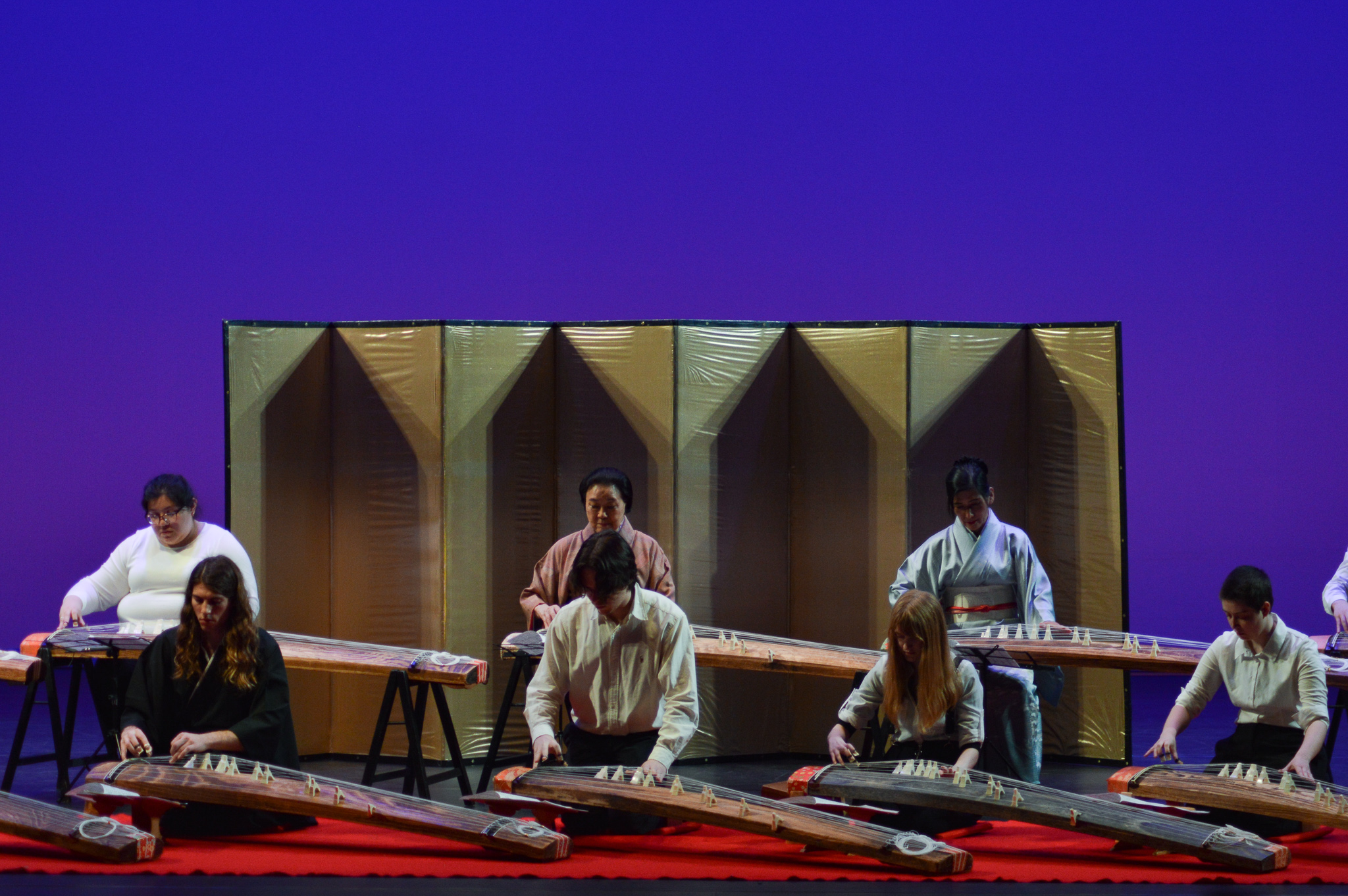This photograph captures a diverse group of seven visible performers, along with a barely visible eighth person, engaged in a musical concert featuring traditional Japanese string instruments likely resembling sitars. The ensemble includes men and women of various races and ages, characterized by differing hairstyles including dark hair, blonde hair, and one woman with very short-cropped hair. The musicians in the foreground are kneeling on a red carpet laid over a black stage floor, playing the long, rectangular string instruments positioned across their crossed legs. Behind them, three performers are seated on stools with their instruments propped up on stands resembling sawhorses. The backdrop of the scene features a purple stage background adorned with decorative screens displaying green, orange, and brown hues with geometric triangular patterns, adding an elegant touch to the setting. This rich and detailed tableau showcases the harmonious blend of cultural artistry in a vivid and colorful stage environment.